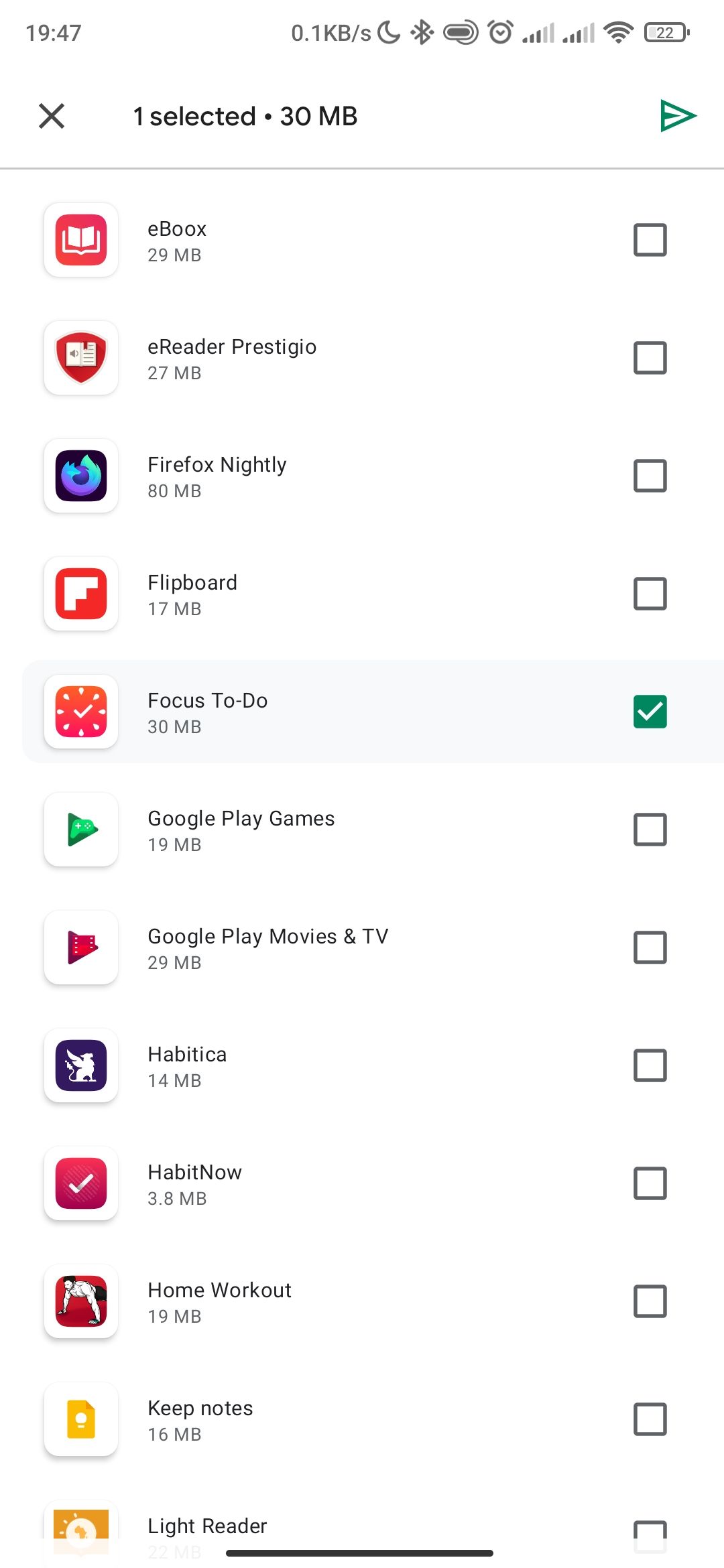The image displays a clean user interface screen, most likely from a mobile device. At the top, standard symbols are visible. Interestingly, where the time is usually displayed on the top left, it instead shows "19:4/". Below this, there's a list of selected applications and their respective storage usage, with one highlighted showing 30 megabytes. The applications listed include:

1. eBooks
2. eReader
3. Prestigio
4. Firefox Nightly
5. Flipboard
6. Focus To-Do
7. Google Play Games
8. Google Play Movies and TV
9. Habitica
10. Habit Now
11. Home Workout
12. Keep Notes
13. Light Reader

Notably, the icon for "Light Reader" is partially obscured, making it unclear if there's more text or an additional word under the visible portion. Each application has a checkbox to its right, except Light Reader, where the checkbox is not fully visible.